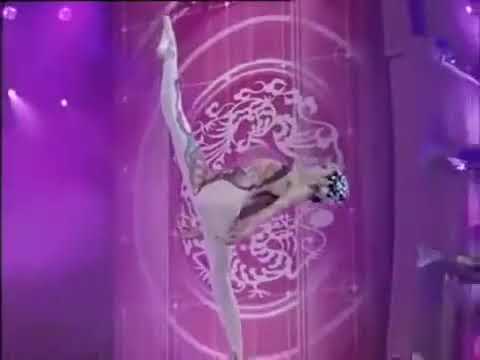The image depicts a somewhat blurry figure of a young female dancer executing a graceful pose. She balances expertly on one leg while her other leg is lifted high, forming a perfect 180-degree angle with her standing leg, almost mimicking a split in mid-air. Her raised leg is nearly vertical, with her foot beautifully extended to align seamlessly with the rest of her leg. The dancer is bent forward, her torso nearly parallel to the ground. She is dressed in a skin-tight gray bodysuit, detailed with white patterns, particularly around the stomach area, accentuating her elegant form. Her black hair is adorned with sparkly green embellishments. The backdrop features a purple curtain adorned with white, lacy decorative elements, including a prominent oval-shaped design at its center, adding a striking contrast to the scene. Small decorative lights dot the left-hand side of the curtain, enhancing the ethereal atmosphere.